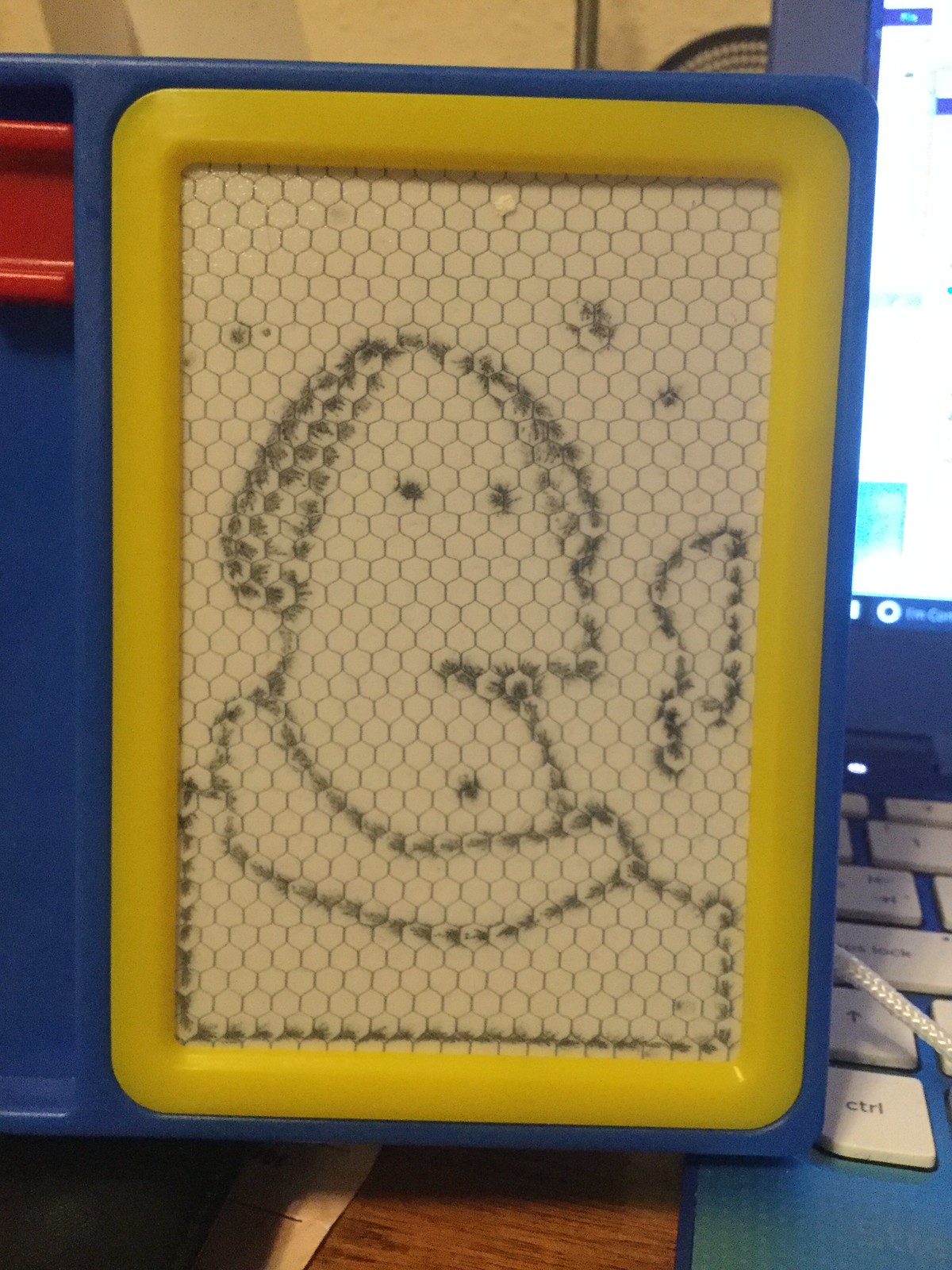This close-up image captures a child's magnetic drawing toy, featuring a blue plastic frame and a yellow-rimmed drawing surface. A whimsical cartoon portrait is sketched on the surface, depicting a person with a pronounced underbite, minimal chin, and short hair. The person appears to be wearing a turtleneck, with simplistic facial details: dot eyes and an understated nose. To the right of the toy, part of a laptop is visible, showing its white keyboard, blue casing, and illuminated screen.